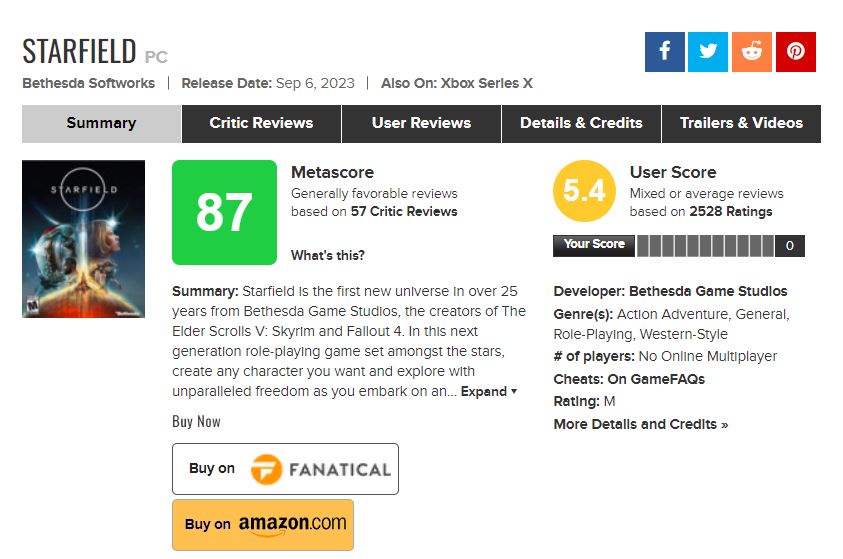Here is a more polished and detailed caption for the image based on the provided voice description:

---

Screenshot of a detailed information page for the PC version of Starfield, an action-adventure role-playing game developed by Bethesda Softworks. Released on September 6, 2023, Starfield is also available on Xbox Series X. The game is a space shooter with RPG elements and has garnered a Metascore of 87 from critics, based on 56 reviews, indicating generally favorable feedback. However, it has a lower user score of 5.4. 

This marks Bethesda Game Studios' first new universe in over 25 years, following their renowned titles like Elder Scrolls V: Skyrim and Fallout 4. Starfield offers next-generation role-playing experiences, allowing players to create any character they desire and explore space with unparalleled freedom.

The summary also lists where the game can be purchased, such as Fanatical and Amazon, and provides additional details regarding its developer, genre, number of players, online multiplayer features, cheats on GameFAQs, and an M (Mature) rating. Further sections on the page include critic reviews, user reviews, game details, credits, trailers, and videos.